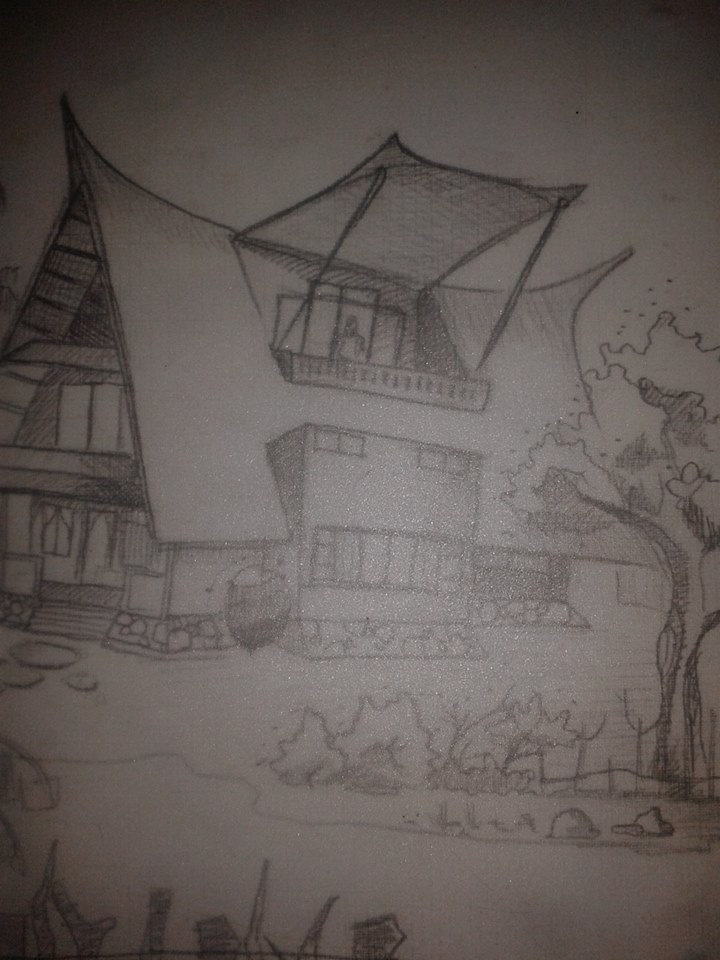A detailed sketch depicts an A-shaped house enveloped in dark shading, creating a somewhat ambiguous image. The structure stands tall with three distinct levels. 

The left side of the image reveals the house's entrance, featuring two windows flanking a door on the ground level. Another window is visible on the second level. At the center of the sketch, the house boasts a large window and a balcony, supported by an awning on both sides. Below this balcony, there is a square section punctuated with multiple windows.

The right side of the scene displays a tree accompanied by clusters of bushes. The bottom left corner of the sketch is adorned with rocks and additional vegetation, all intricately detailed in shades of gray, black, and white.